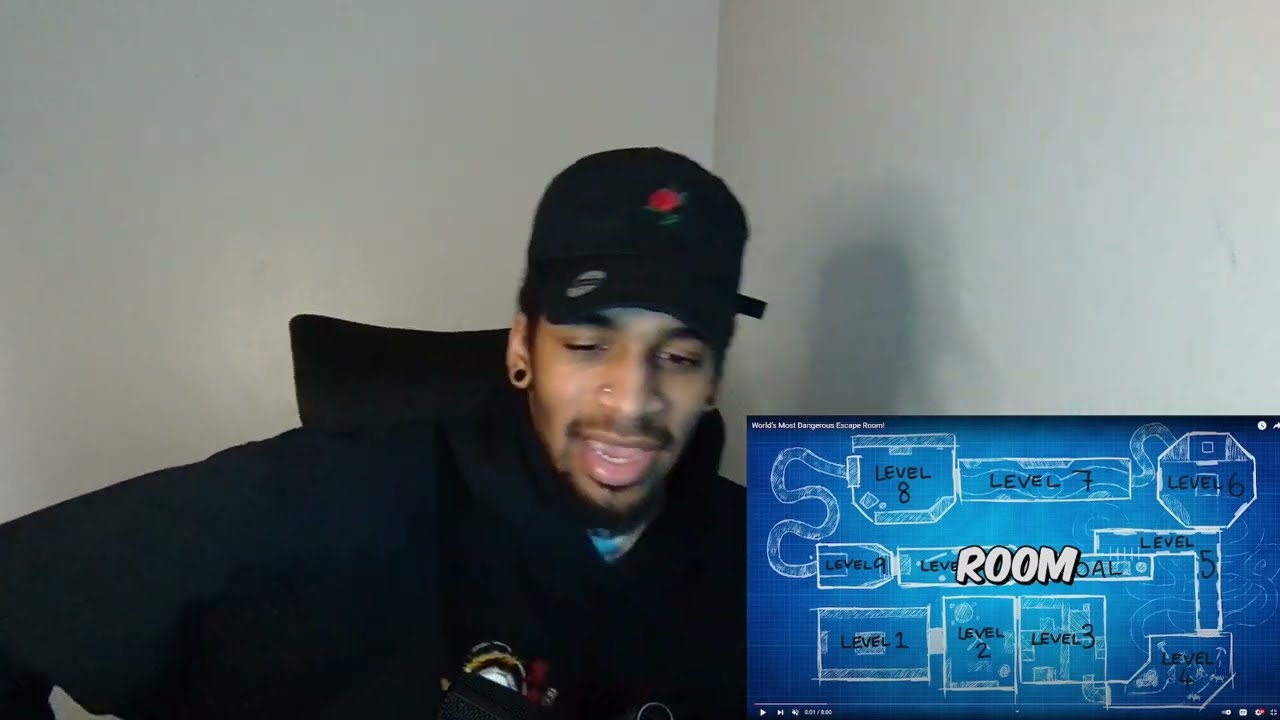The image features a young African American man wearing a black hoodie and a black baseball cap adorned with a red rose logo and green detailing. He has black gauges in his ears and a mustache. The setting appears to be a room with white walls, where shadows indicate he's positioned near a corner. He is seated in a black chair with a headrest, possibly engaging in a live recording or Zoom meeting. On his monitor in the lower right corner of the image, there is a graphic titled "World's Most Dangerous Escape Room." The screen displays a blueprint-like map consisting of various interconnected rooms labeled from Level 1 to Level 9, depicted in a maze-like format. The word "ROOM," in bold white capital letters with a black border, is prominently displayed in the center of the on-screen graphic. It appears he is reviewing or discussing the escape room game, providing his thoughts and commentary.